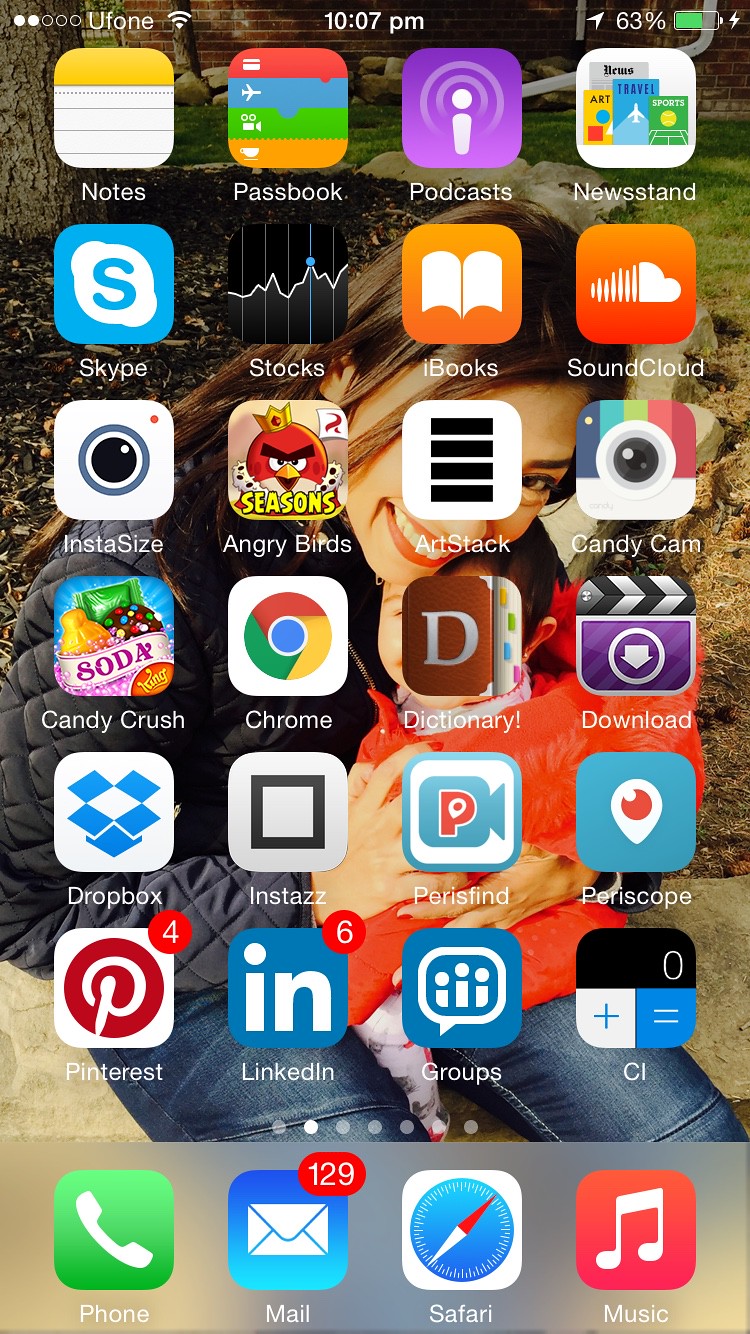The front screen of a smartphone showcases various elements with a high level of detail. At the top, the screen displays "Uphone" in white letters, along with the signal strength icon, also in white. Adjacent to it is the time "10:07 p.m.," a small white arrow, and the battery percentage showing "63%."

The focal point of the screen is a heartwarming image of a woman and her baby. The woman, with long dark hair, wears a dark-colored jacket and blue jeans. She holds a baby dressed in a little orange outfit close to her chest, and she appears to be slightly bent over.

Surrounding this image are numerous app icons including Notes, Passbook, Podcasts, Newsstand, Skype, Stocks, iBooks, SoundCloud, Instasize, Angry Birds, RStack, Candy Cam, Candy Crush, Chrome, Dictionary, Downloads, Dropbox, Instant, Paris Find, Periscope, and Pinterest. Some apps display notification badges: a red circle with the number four on one app, and another red circle with the number six on LinkedIn. Additional apps include Groups and CI.

At the bottom of the screen are key functional icons: Phone, Mail (showing 129 unread emails), Safari, and Music.